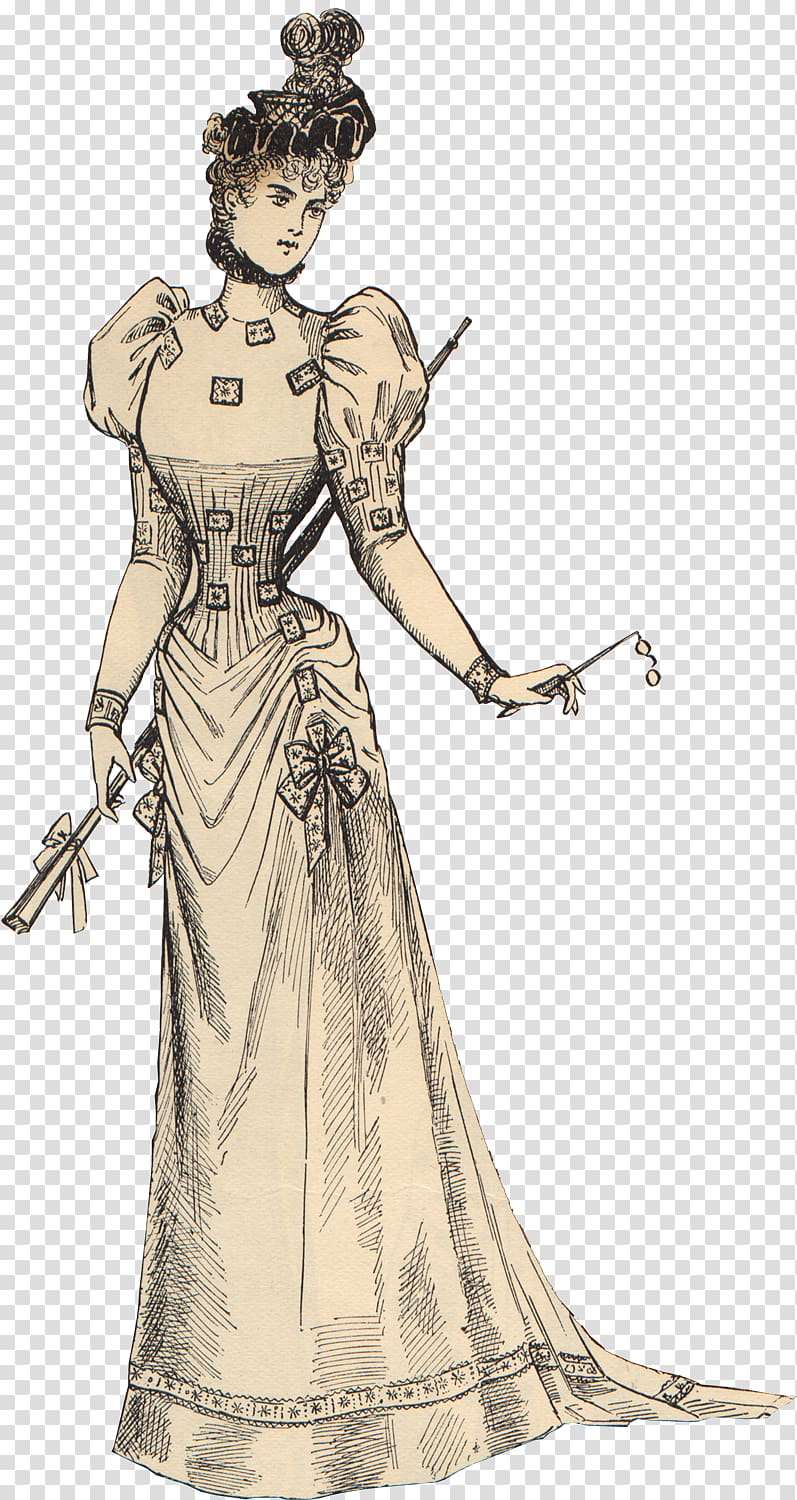This detailed black and white illustration features a beautifully dressed woman in a vintage, potentially Victorian-inspired outfit. The woman stands out prominently against a photoshopped checkerboard background, indicating it's a transparent PNG image likely used for design purposes. She wears an elaborate dress with puffy shoulders, a tight corset, and a high neck, complemented by intricate embellishments such as a ribbon design near her hips and detailed patterns at the hem of her flowing skirt. 

Her hair is styled in an elegant, large bun topped with a frilly hat adorned with a flower or ribbon. In her right hand, she holds a parasol, its handle visible near her hand while the rest extends behind her. Her left hand clutches a pair of opera glasses, enhancing the vintage feel of the portrait. The overall style suggests an antique illustration but likely created with modern graphic tools, giving it an appearance of an old photograph on aged paper. This descriptive and atmospheric image could serve well in story-driven game design or other creative applications.